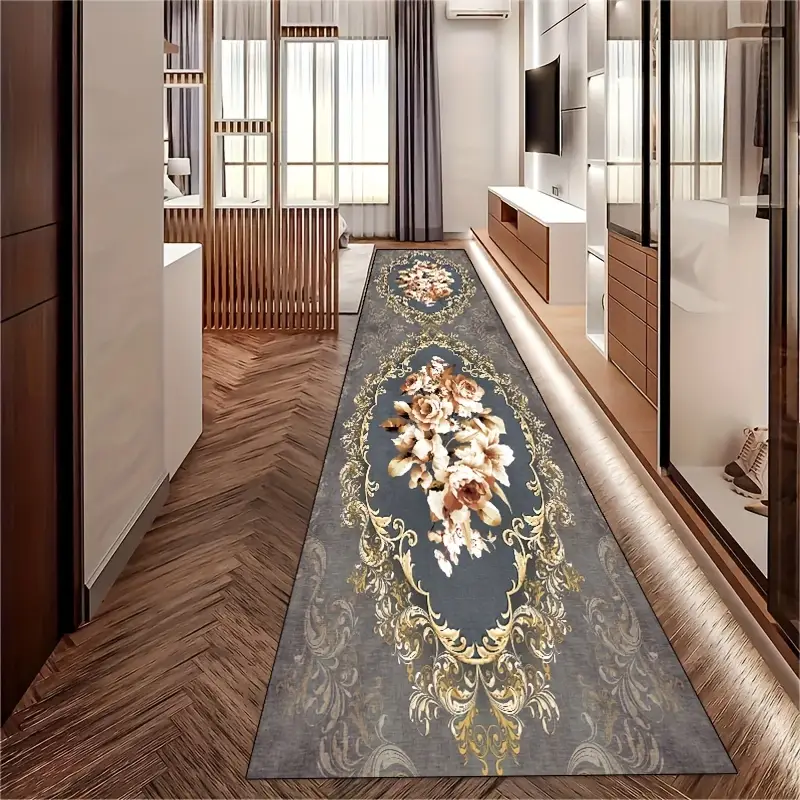The image depicts a sophisticated interior that likely belongs to a high-end home or a showcased design from an interior design catalog. The floor is a distinct brown surface that might be hardwood or linoleum, extending across the room and appearing to curve upward towards the wall on the right side, suggesting either an optical illusion or unique architectural design. A grey carpet with floral designs in green, white, and brown runs along this floor, enhancing the room's elegance.

On the left side, a chocolate brown door is partially visible, leading into a space with white walls. Adjacent to the door is a countertop, seamlessly transitioning into the room’s layout. Also visible on the left are window-shaped cutouts in the wall, offering a view into an adjoining bedroom. This bedroom features a white bed with matching cushions and bed sheets, flanked by a night lamp and illuminated by natural daylight streaming through a glass window adorned with long grey curtains.

On the right side of the image, there are several home furnishings, including a white dresser with brown front panels and a flat-screen TV mounted on the wall above it. Below the TV, the dresser has a spacious bottom drawer and two smaller upper drawers. A wardrobe with glass panes stands nearby, revealing shoes on the bottom level and hanging clothes above. There are shelves and a closet in the right corner, emphasizing the room's practical and aesthetic elements. An AC unit is positioned on one of the white walls, indicating the room’s modern amenities.